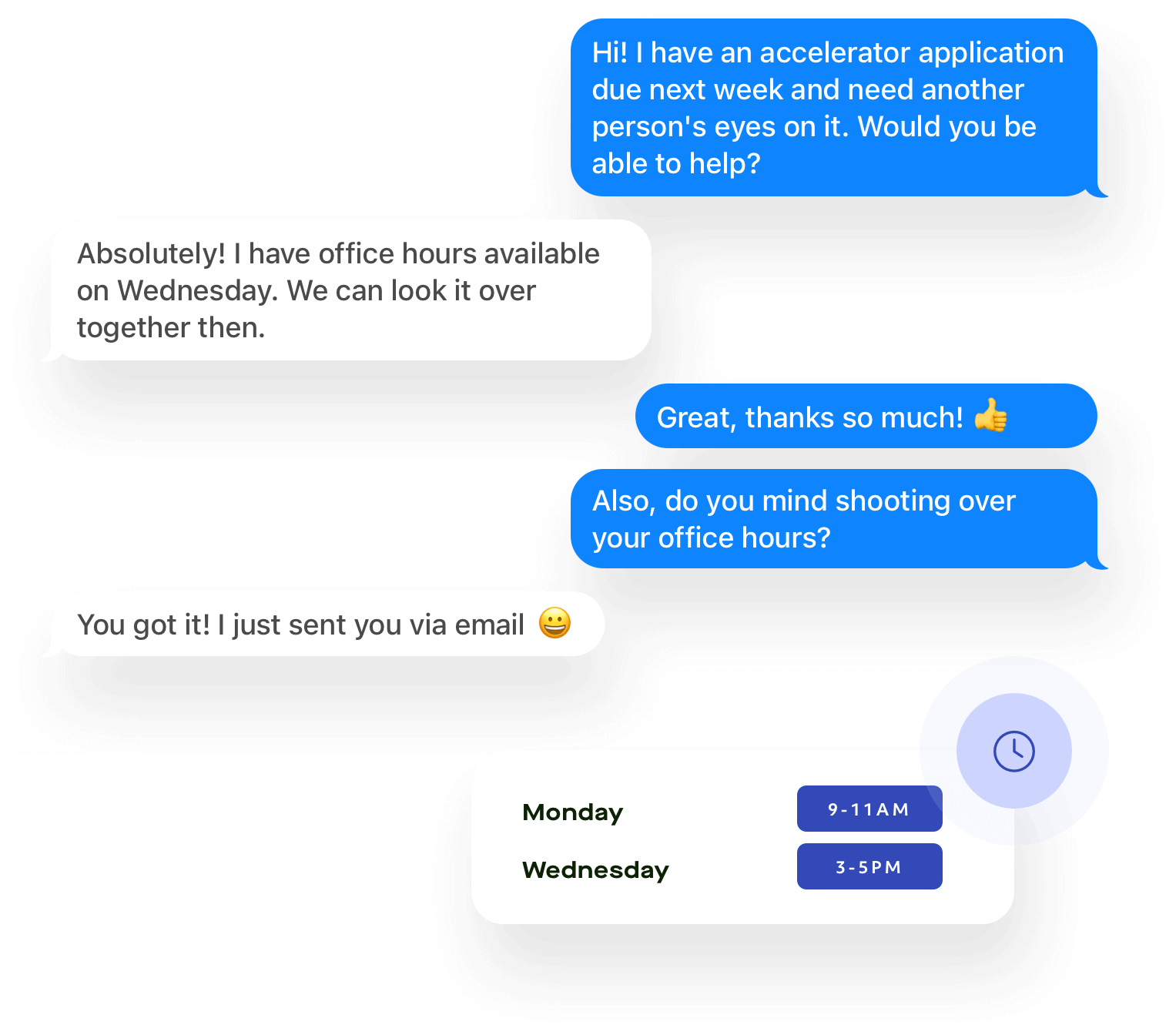A screen capture image of a chat conversation shows Person A requesting assistance with an accelerator application due next week. Person A sends a message saying, "Hi, I have an accelerator application due next week and need another person's eyes on it. Would you be able to help?" Person B responds affirmatively, stating, "Absolutely, I have office hours available on Wednesday. We can look it over together then." Person A expresses gratitude with a "Great, thanks so much," followed by a thumbs-up emoji. Person A then asks, "Also, do you mind shooting over your office hours?" Person B reassures with, "You got it," and adds that they have sent the schedule via email, including a smiley face emoji. The chat also includes a small graphic that lists Person B's available office hours as Monday 9 to 11 AM and Wednesday 3 to 5 PM, which seems to have been shared from a calendar program.